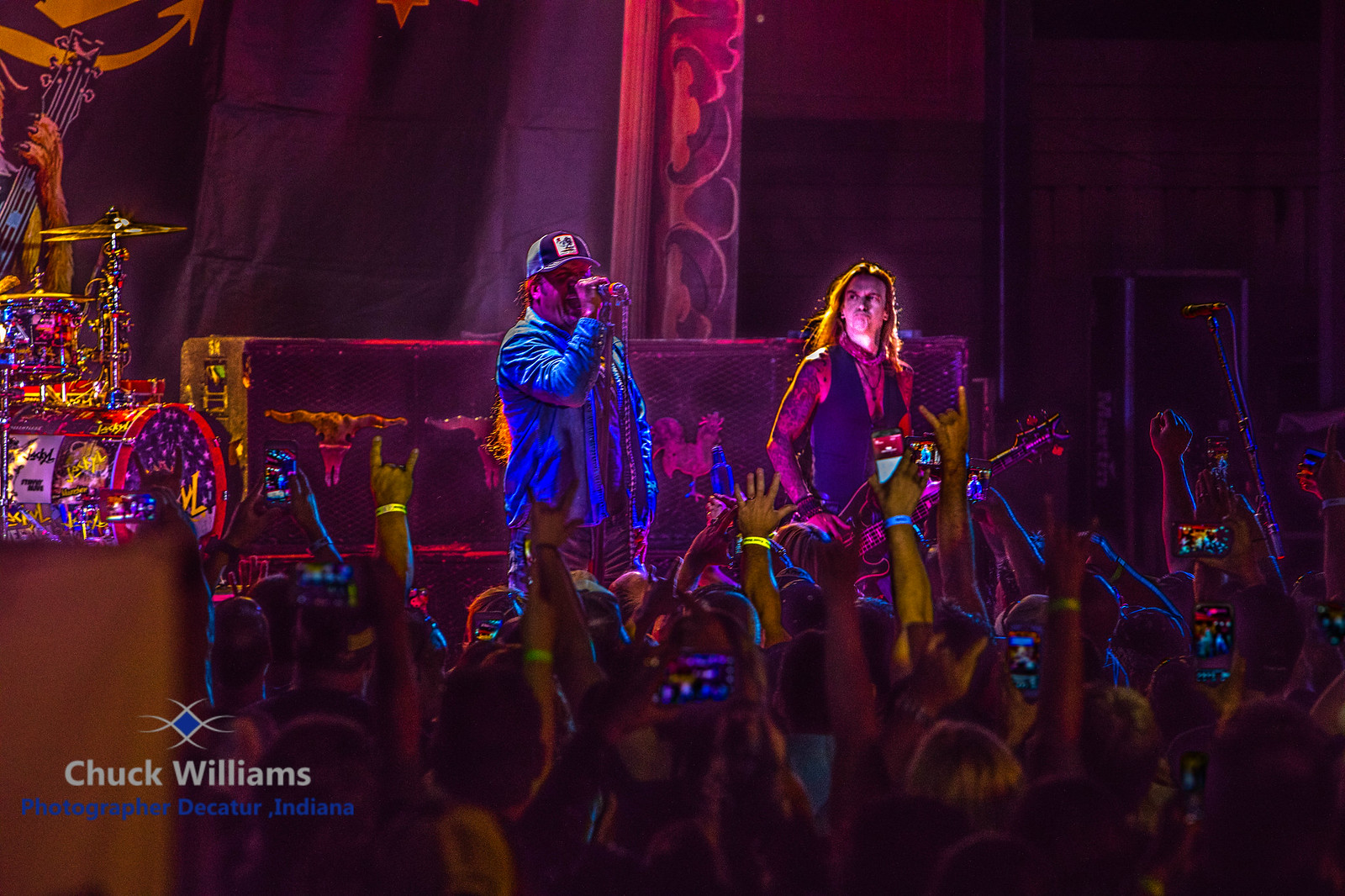This photorealistic image, likely a painting rendered over a photograph by Chuck Williams, a photographer from Decatur, Indiana, depicts an indoor concert scene with crowds gathering near the stage, enthusiastically throwing up signs and sporting blue and yellow wristbands. On stage are two distinct musicians: on the left, a rapper with a long ponytail, baseball cap featuring a logo, blue jacket, and blue jeans is singing into a microphone. On the right, a rock star with completely tattooed arms and chest, a necklace, long dark brown hair, and a black vest without a shirt is immersed in playing a black guitar. To the left, the drum kit and speakers add depth to the vibrant, dark stage illuminated by purplish lights. Text in the bottom left corner reads "Chuck Williams Photographer, Decatur, Indiana."